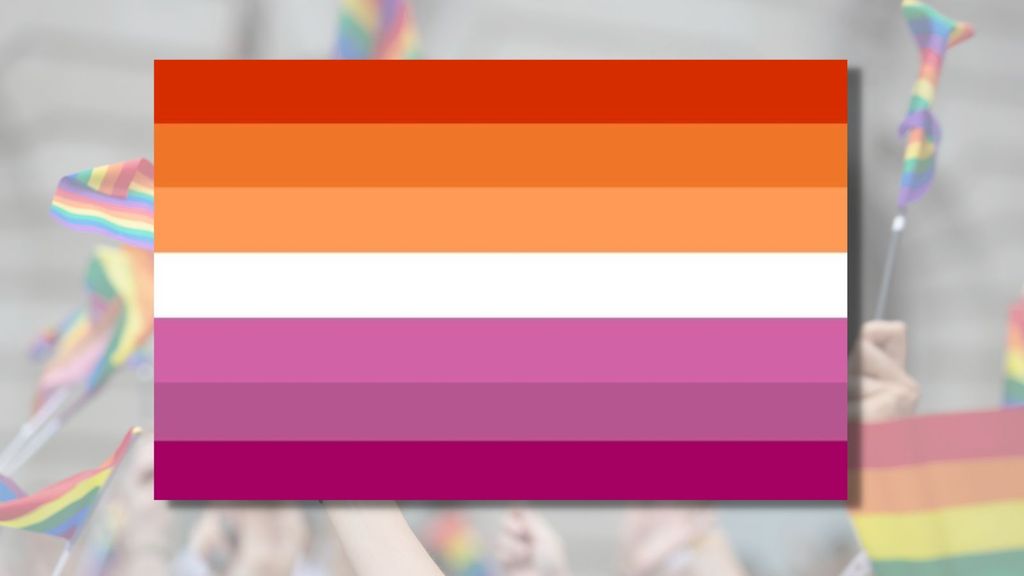The image features the Lesbian Pride flag, characterized by seven horizontal stripes in a gradient from dark burnt orange at the top to dark plum at the bottom, with colors transitioning through various shades of orange and purple, and a central white stripe. Specifically, the stripes progress from dark burnt orange, orange, light orange, white, light purple like plum, deeper plum, to a dark plum color. The top three stripes are shades of orange and pale, the middle stripe is white, and the bottom three are purple tones increasing in darkness. The background of the image displays additional rainbow pride flags being held and waved by people, suggesting it was taken at a pride event. The scene showcases a vibrant celebration of LGBT identities, with numerous hands and arms holding and waving colorful ribbons and flags.